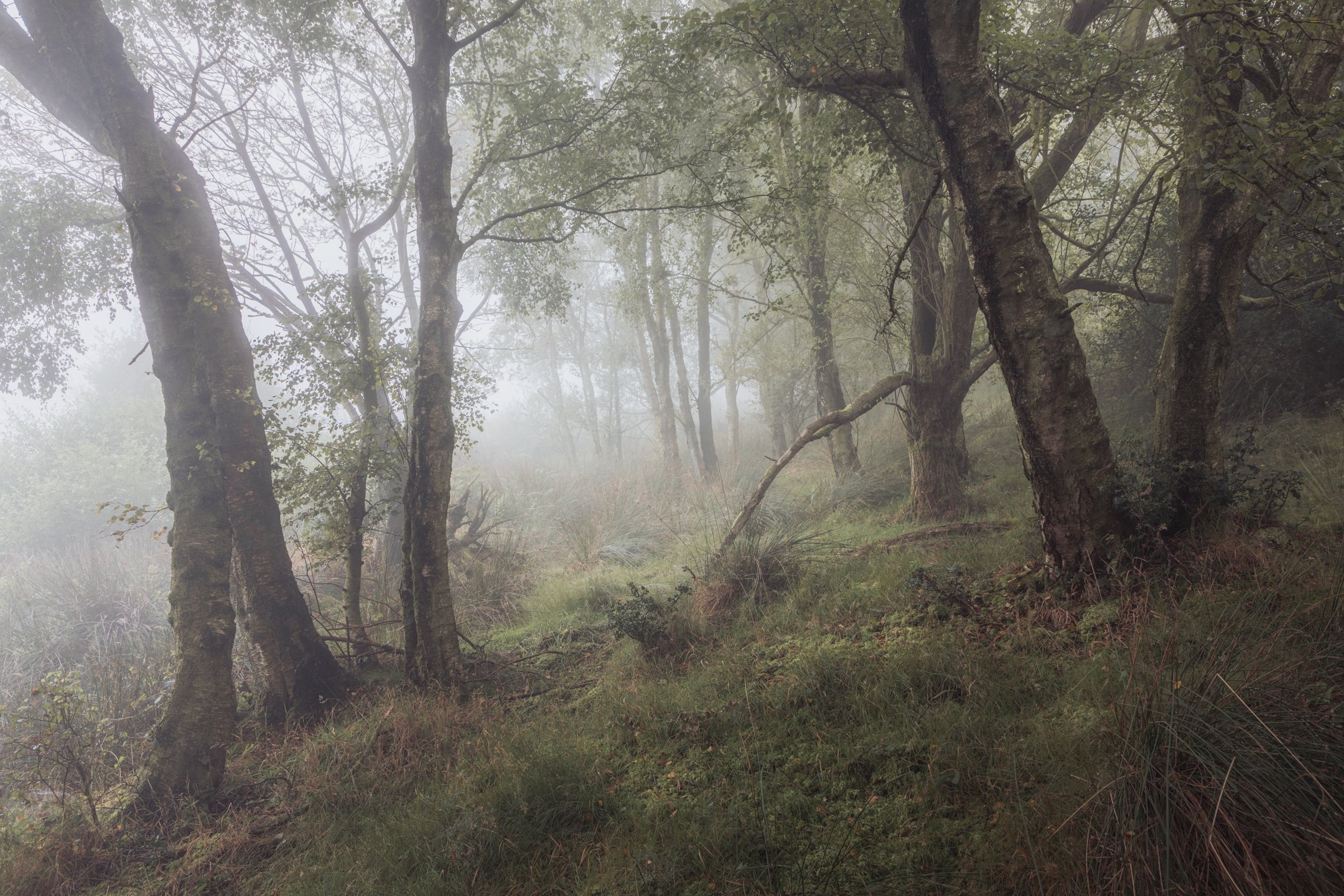In this photograph taken outside, we observe a forest scene shrouded in a dense mist or fog, creating an eerie and mystical atmosphere. The forest is situated on a slight incline, with the right side of the image showing a higher elevation than the left, suggesting a descent as our eye moves across the frame. The forest floor is lush with green vegetation, although some plants exhibit a yellowish tinge, possibly from a lack of water. Wild grass and small bushes sporadically cover the ground, interspersed among the numerous trees that dominate the scene. 

These trees, some old and weathered, stretch upwards with both leafy branches and some bare limbs, contributing to a somewhat rugged landscape. Notably, there is a large broken branch to the right; while still attached to the tree at its base, it has fallen and rests on the ground. The lighting in the photograph is dim and subdued, heavily influenced by the overcast sky and pervasive fog, which also obscures the view into the distance, revealing only more trees veiled in mist. The entire scene lacks a clear pathway, emphasizing the untouched and natural essence of this forested hillside.